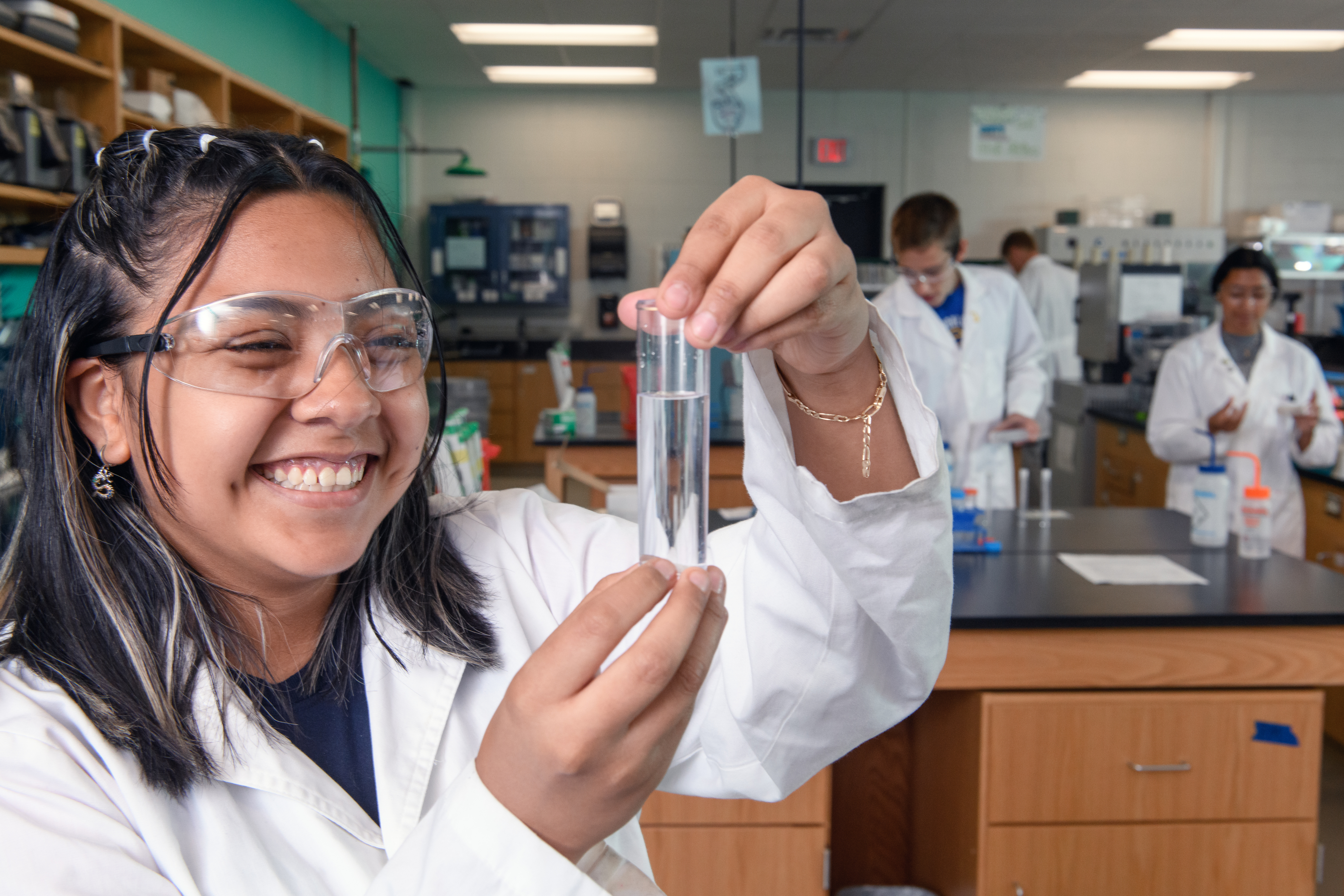In the photograph, a group of high school students is working diligently in a science lab, all clad in white lab coats. The focal point on the left-hand side features a teenage girl with medium-length, dark brown hair with lighter highlights, styled into small, sectioned ponytails using elastics. She has dark hair and tan skin, accentuated by clear safety goggles and a blue shirt peeking out from under her lab coat. Smiling, she holds a small beaker with a clear liquid, possibly water, with both hands. The background reveals more students engaged in various experiments, surrounded by typical lab equipment and desks, suggesting a lively and educational laboratory environment. The detailed setting, their attire, and the focused expressions reflect an immersive learning experience in science experimentation.